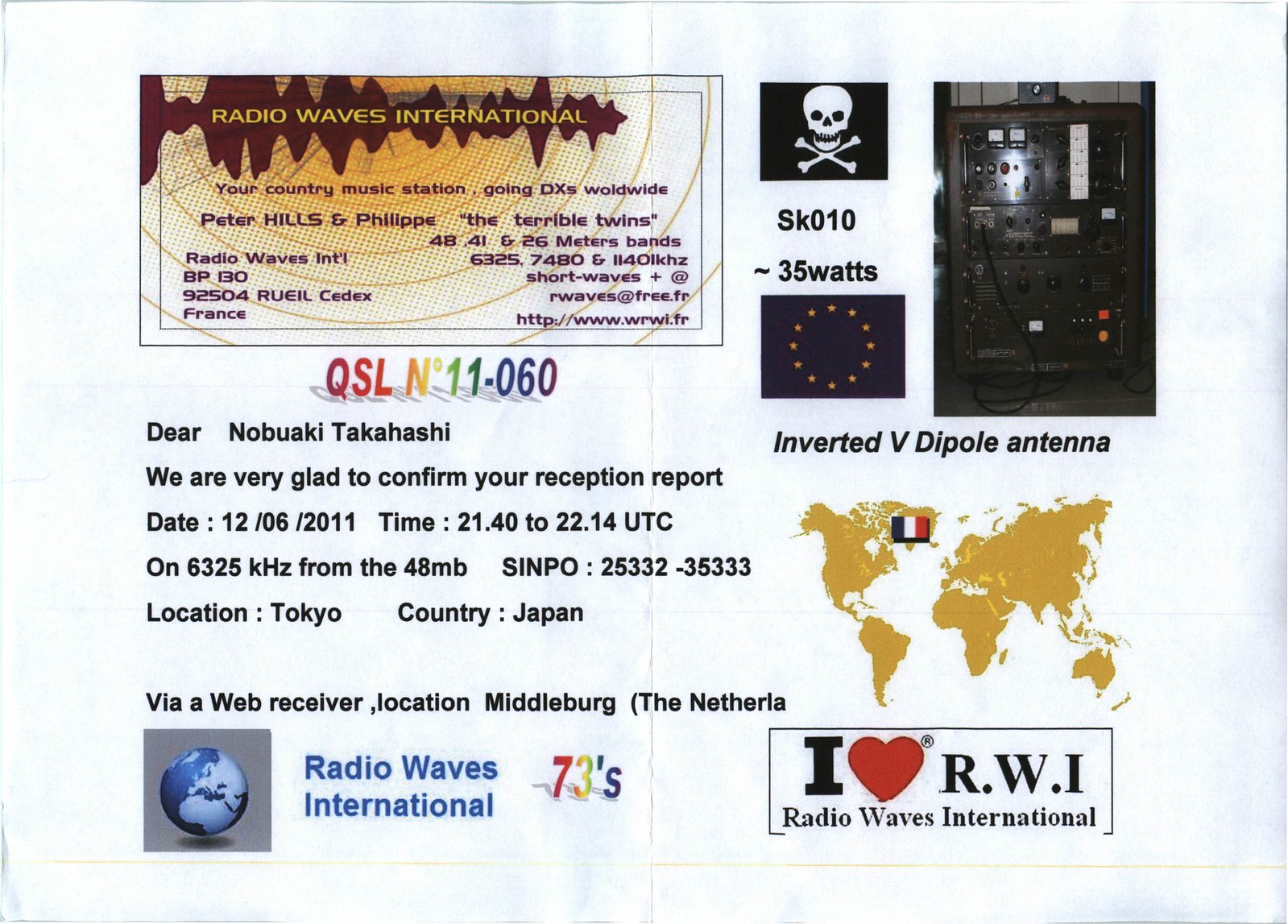The image is a vibrant QSL card from Radio Waves International, designed in a full-color print. It features a multitude of colors including blacks, whites, browns, yellows, reds, blues, grays, greens, purples, and oranges. The top of the card prominently displays "Radio Waves International, your country music station, going DX worldwide," along with contact information for the station and their website, http://www.wrwl.fr. In the upper right-hand corner, there's a photograph of a piece of shortwave radio equipment. Next to it, there are two flags: a skull and crossbones flag and a blue flag with a circle of yellow stars. Below these, a brown map of the world is displayed with an Italian flag curiously placed over Greenland. Directly under this map, there's text stating "I heart RWI, Radio Waves International."

The card confirms the reception report of a listener, Nobuaki Takahashi, outlining the reception details: date 12-6-2011, time 2140 to 2214 UTC, on 6325 kHz from the 48MB, with SINPO code 25332-35333. The listening location was Tokyo, Japan, via a web receiver located in Middelburg, The Netherlands. Additionally, technical specifications of the transmission—like the 35 watts output and inverted V dipole antenna—are noted. In the lower-left corner, there's a blue globe labeled "Radio Waves International 73s." The card is signed off with "73s," a term signifying "so long" in ham radio jargon, and an image of a heart symbolizing love for Radio Waves International.